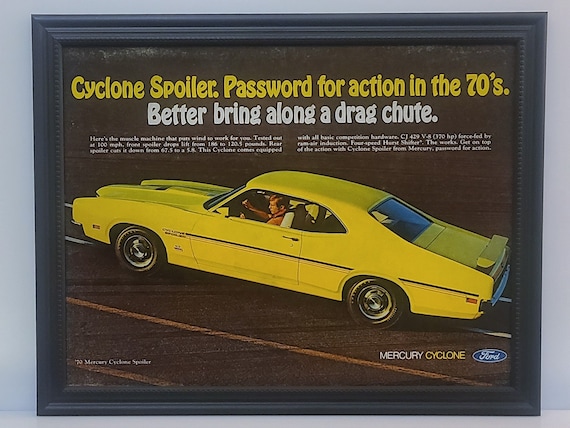The image depicts an advertisement, likely from the 1970s, framed in a black wooden beveled edge and positioned against a greyish-bluish wall on a white surface. The poster has a dark brown background, prominently featuring a mustard-yellow sports car tilted upwards diagonally towards the top left corner. The car, identified as a Mercury Cyclone, is detailed with a black stripe running along its body from the front wheel arch to just before the rear. The car's black tires are accentuated with silver rims. Inside, a man with dark brown hair, wearing a light brown shirt, is seen gripping the steering wheel. Across the upper section of the poster, bold yellow text reads "Cyclone Spoiler, password for action in the 70s." Below this, in white text, it says "Better bring along a drag chute." The lower portion includes unreadable small white text arranged in two columns of three lines each. In the bottom right, the Ford logo with the word "Ford" in italics is displayed, alongside white text that reads "Mercury" and "Cyclone." Overall, the advertisement showcases the Mercury Cyclone as a vehicle synonymous with thrilling action from the 70s.